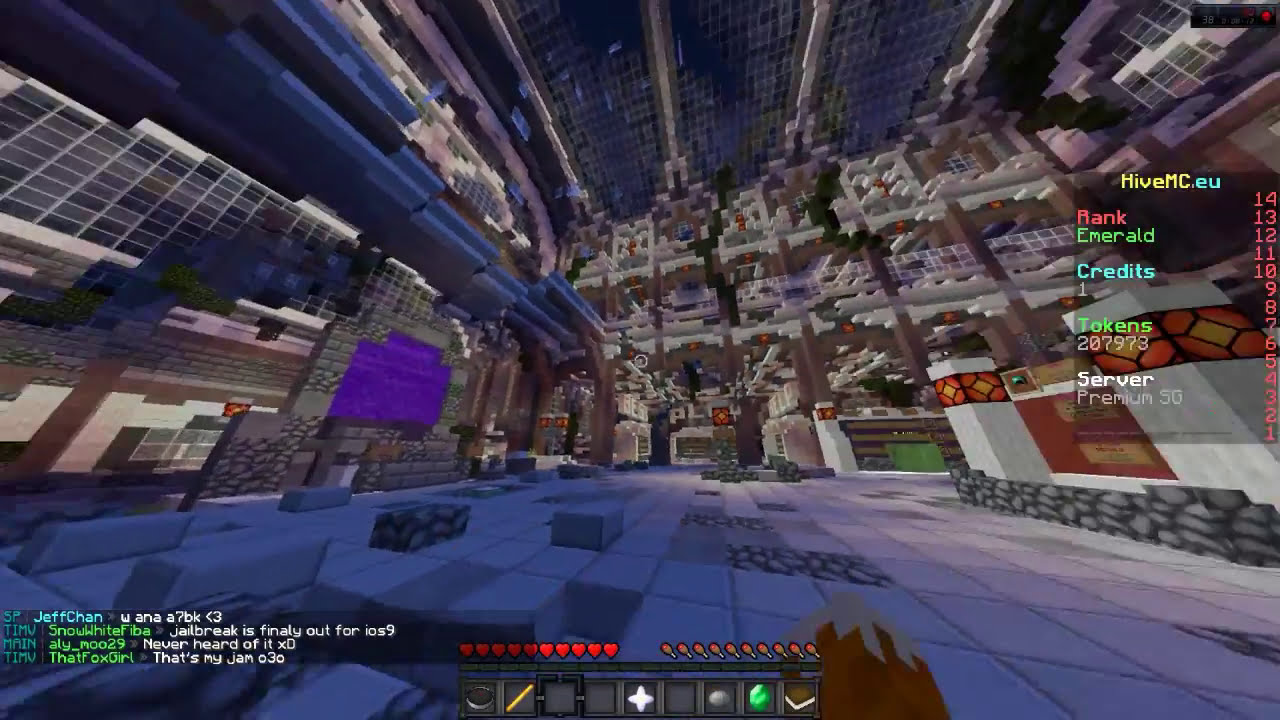The image appears to be a screen capture from the video game Minecraft. The perspective is from a high vantage point, possibly at the edge of a skyscraper, looking down at a cityscape composed of smaller buildings and blocks, evoking a sense of vertigo. Visible on the right side of the screen is an informational menu with the text "hivemc.eu" at the top, followed by categories such as Rank: Emerald, Credits: 1, Tokens: 207,973, and Server: Premium 5G. In the bottom left corner, there's an ongoing chat conversation featuring users like Jeff Chan, Snow White, Feeba, Allie, Moo29, and ThatFoxGirl. The bottom edge of the screen displays a row of player-relevant icons, including red hearts indicating lives, and various items like a silver ring, brown stick, white plus sign, green gem, brown book, and a circular gray stone. The overall scene suggests a detailed Minecraft environment with a mix of towering skyscrapers and intricate block structures.